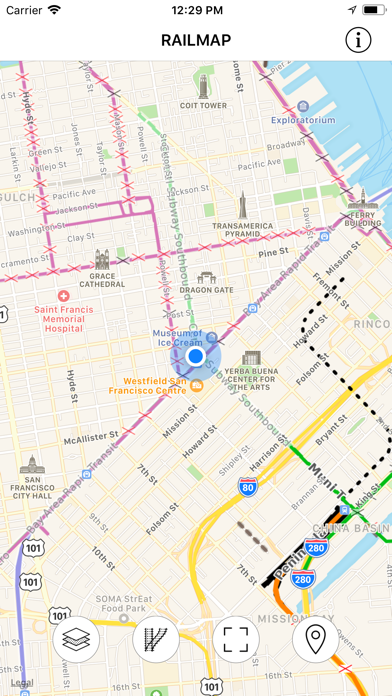This detailed caption provides a thorough overview of a screenshot from the RailMap application:

---

Screenshot of the RailMap application, showcasing its utility in navigating the rail networks of San Francisco. The upper left-hand corner displays several key interface elements: a “Carrier” label next to three signal bars, a time marker reading “12:29 PM” in the center, a directional icon, and a battery indicator showing approximately 75% charge. The title "RailMap" is prominently displayed, and on the upper right-hand side, there is a lowercase 'i' inside a circle, likely an information icon.

Below this top bar, the screen reveals a detailed city map, closely resembling Google Maps. Various San Francisco landmarks are notably marked, including Coit Tower, Grace Cathedral, San Francisco City Hall, Yerba Buena Center for the Arts, the Ferry Building, and the Transamerica Pyramid. These points of interest help in orienting and confirming the map's coverage area.

The map is densely overlaid with multiple lines in different colors and patterns representing various routes. Yellow street lines distinguish the regular roadways, with thicker yellow lines highlighting major highways like Highway 80 and 280. Pink lines adorned with X marks, as well as blue and black dotted lines, and other lines featuring purple and pink X's, indicate different railways and possibly their stations or significant points.

A special notation on one of the pink lines reads "BART Area Rapid Transit,” denoting a segment of the Bay Area Rapid Transit network. These detailed notations and colored routes illustrate, though possibly unclear in specificity, the extensive rail infrastructure.

A blue beacon with a central white circle and an encompassing translucent larger blue circle marks the user's current position, providing a clear point of reference within the expansive map layout.

---

This caption effectively conveys the specifics of the image while incorporating comprehensive details about the visual elements and their significance.